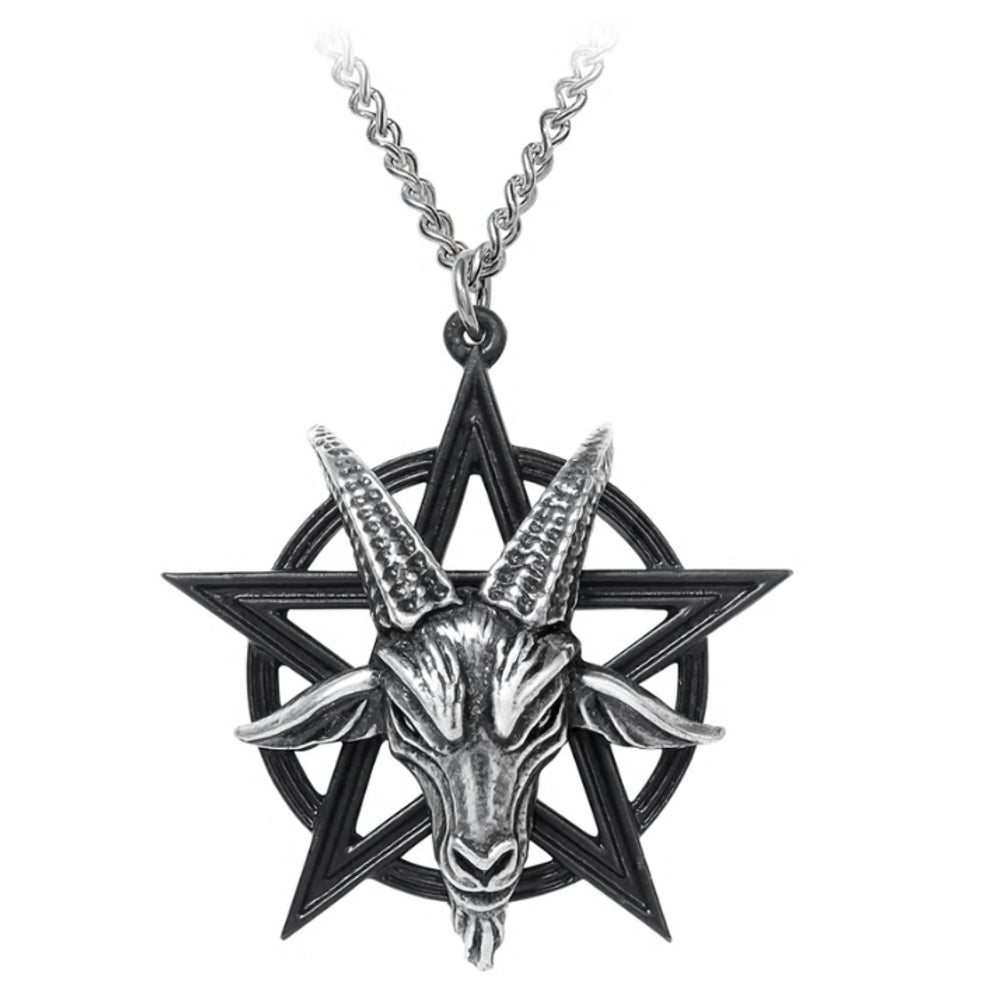The image depicts a pendant necklace set against a completely white background. The necklace chain, composed of small, metallic, silver-colored links, forms a classic chain-link pattern both at the top and bottom. Attached to this chain is a dark, circular pendant. Within the circle is a black star, and overlaid on the star is the detailed depiction of a goat's head, known as Baphomet. The goat has distinctive, tall horns adorned with several rows of black dots on each side, extending all the way up. Its slanted eyes give off an angry expression, and it features a white and gray beard at the bottom. The ears of the goat stick out to the sides. The entire pendant design, combining the dark circle, black star, and the sinister goat's head, conveys a strong association with evil and satanic symbolism, rendered in shades of black, gray, and light gray.